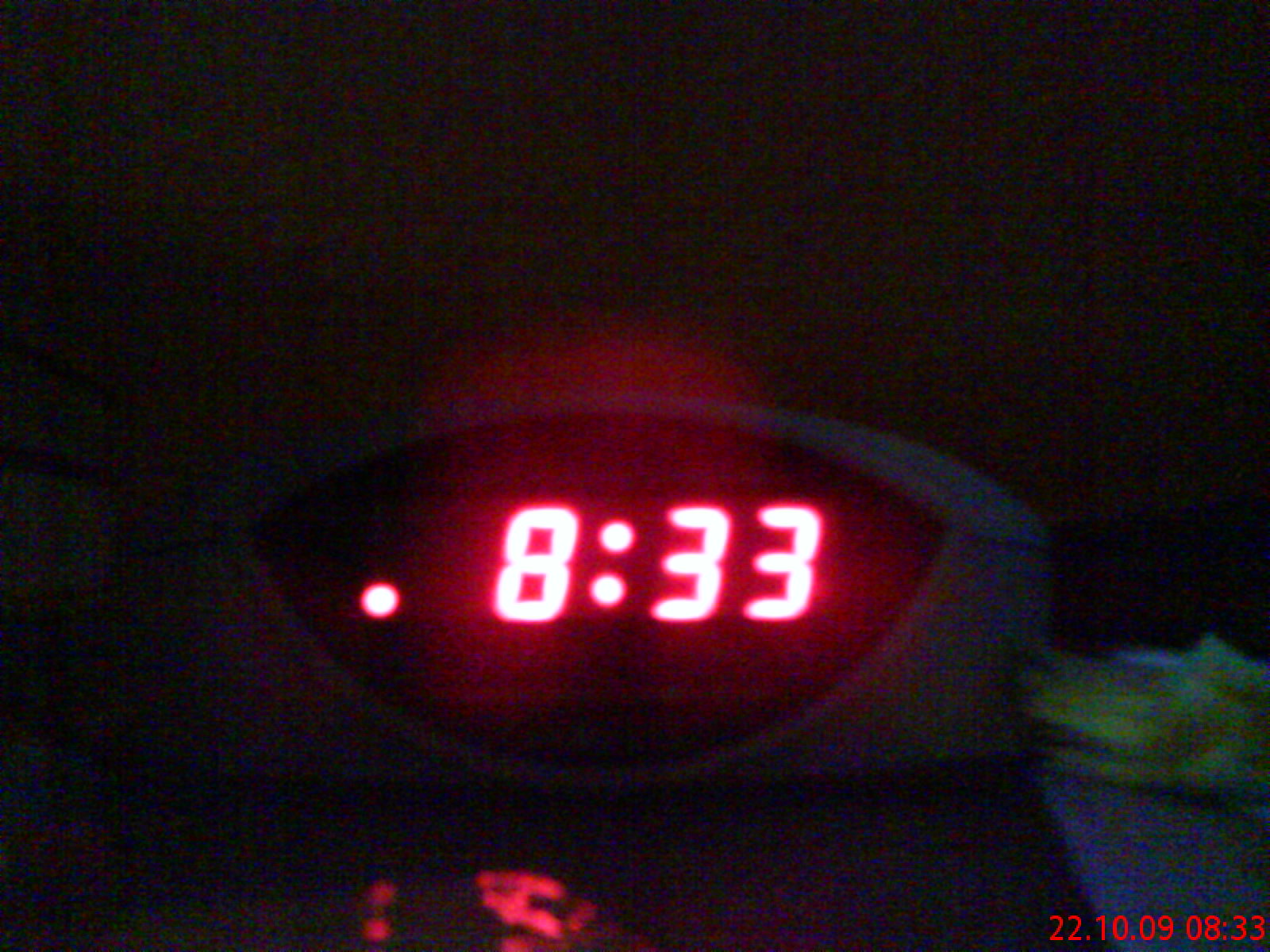In this grainy, low-resolution photograph—likely captured with a 1980s-era camera—a vintage white alarm clock occupies the center of the image. The clock, reminiscent of a smiling open mouth due to its shape, features an LED display with a deep red background. The display reads "8:33 PM," as indicated by the illuminated dot at the bottom left of the numbers. Surrounding the LED display are numerous red pixels, contributing to the overall glow.

The background is indeterminate, appearing as a light-colored wall or surface, while on the right side of the image there's a small item that resembles a bowl of chips. At the bottom of the photograph, there are numbers "22.10.09" and "08.33," suggesting the picture was taken on October 9, 2022, or possibly September 10, 2022, at 8:33 PM.